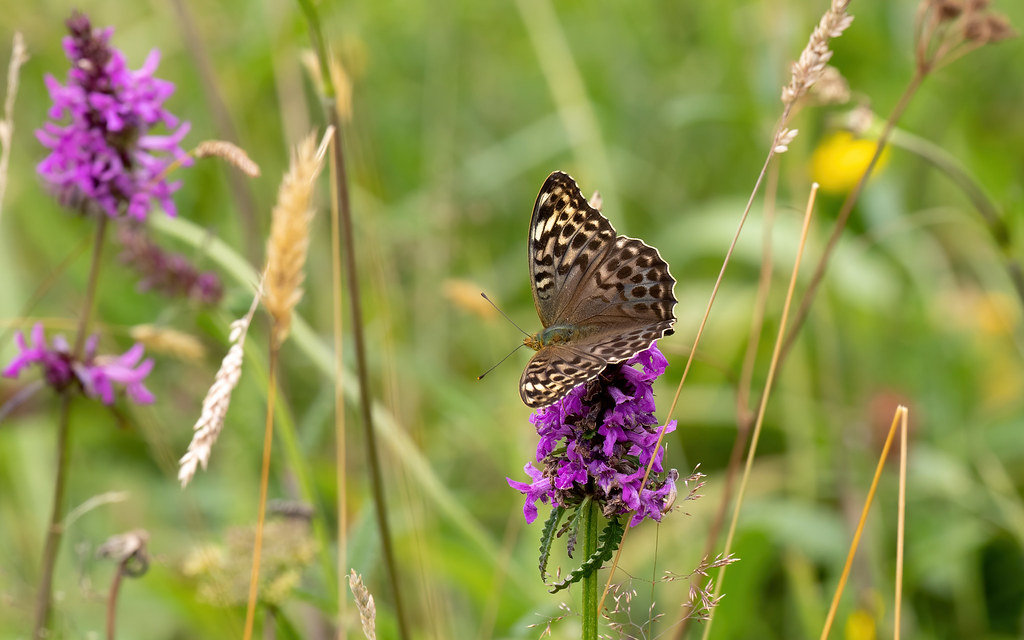In a lush, blurred green background, a detailed landscape-oriented photograph captures a breathtaking natural scene. At the center of the image, perched on a cluster of light lavender flowers with dark purple bases, rests a striking butterfly. The butterfly's wings are slightly spread open, showcasing a light cream-yellow coloration with black borders and black dots, creating a tiger-eye effect. Its bluish-brown elongated body aligns horizontally across the flower, with its head facing left and its tail right. The butterfly's two long antennae extend elegantly from its head.

To the left of the central flower stalk, a brown wheat stem with a wheat spike at the top adds an earthy contrast. Additional purple flowers, similar to the central cluster, can be seen blurred in the background, alongside a hint of a small yellow flower on the right. The overall ambiance suggests a natural, serene setting, possibly captured by a keen photographer aiming to highlight the delicate interplay of flora and fauna.